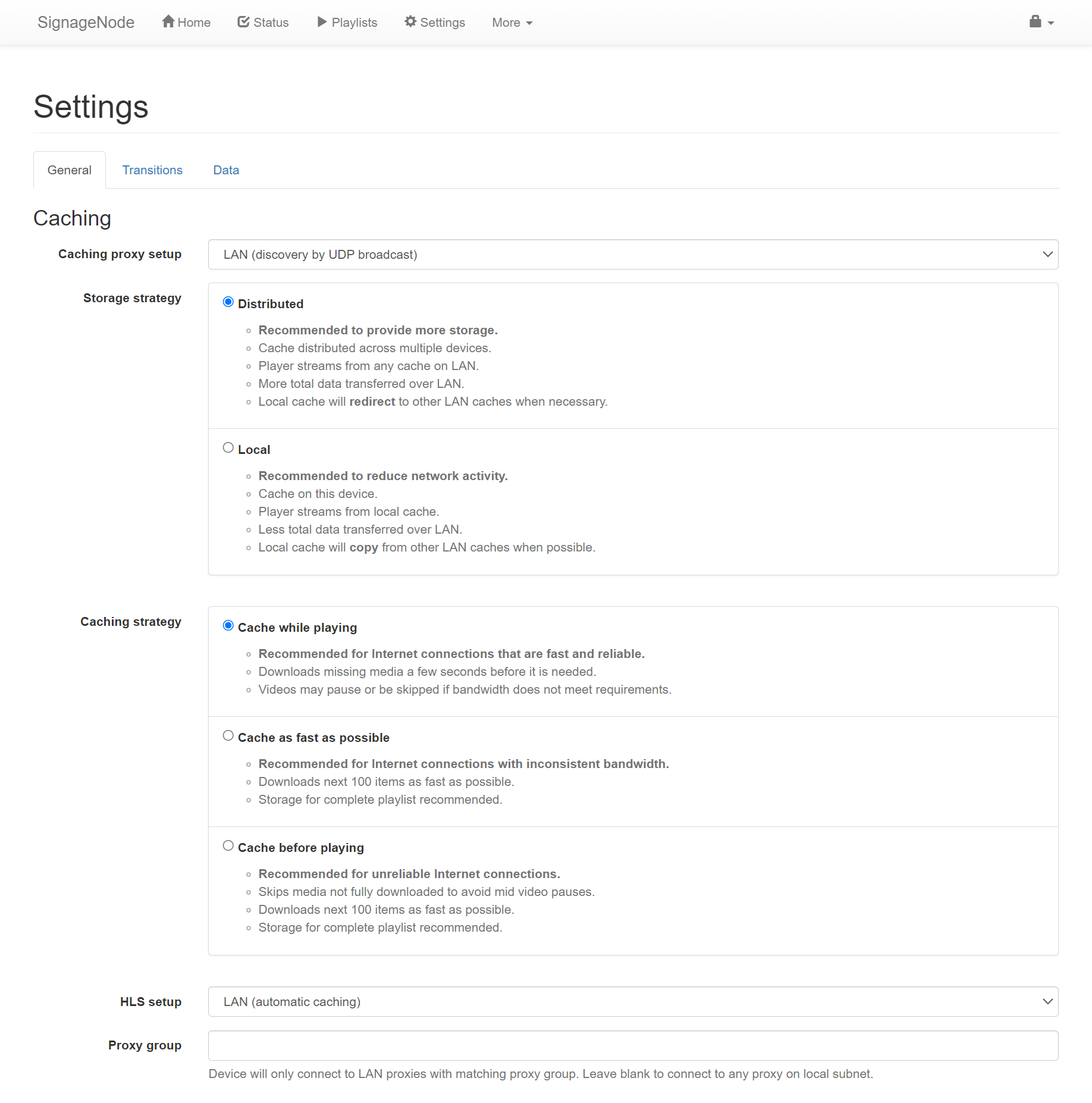This image depicts the settings page of a website belonging to a company called SignageNode. The company's name, "SignageNode," is prominently displayed in the upper left-hand corner of the page. Adjacent to the name are several navigation buttons arranged in a row: Home, Status, Playlists, Settings, and a dropdown menu labeled "More." Additionally, a shopping cart icon with a dropdown menu is located in the upper right-hand corner.

Directly below the company logo is the section title "Settings," which is written in black font against a white background. The settings section is divided into three tabs: General, Transition, and Data. The "General" tab is currently active, highlighted by black text, while "Transition" and "Data" are shown in blue text, indicating they are inactive.

Within the General tab, the first subsection is labeled "Caching." This section includes various configuration options:
- "Caching Proxy Setup"
- "Storage Strategy" with a dropdown menu to select LAN discovery via UDP broadcast
- Two radio button options labeled "Distributed" and "Local," with "Distributed" currently selected.

Following the Caching Proxy Setup is the "Caching Strategy" category, offering three options for caching behavior:
- "Cache While Playing" (currently selected)
- "Cache as Fast as Possible"
- "Cache Before Playing"

Each of these settings is clearly delineated, allowing users to tailor the website's behavior to their specific needs.